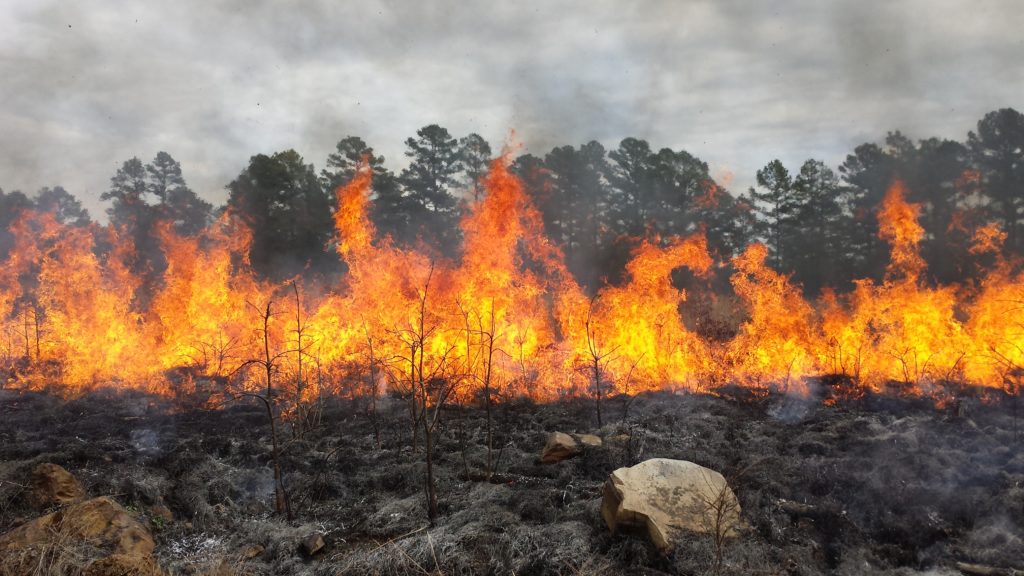The image captures a potentially unsettling, yet strangely orderly, scene of a controlled forest burn. The landscape is divided almost precisely along a straight charred line, giving an impression of calculated deliberation. Dominating the middle section of the rectangular photograph are formidable flames, several feet high, appearing to progress methodically in a line. The fire's hues—golden yellows and oranges—lend a fierce contrast against the dark, smoke-heavy sky that envelops the top part of the frame. To the foreground and the lower part of the image, the ground is visibly blackened with charred twigs and brush sparsely protruding from the blackened soil. The landscape ahead is stark and barren, speckled with some light beige and gray rocks nestled in black soot. In the background, a thin line of tall deciduous trees stands incongruously green, though they are on the brink of being engulfed by the formidable flames. The overall atmosphere is both frightening and fascinating, marked by the orderly nature of the flames despite the inherent chaos that fire generally brings.